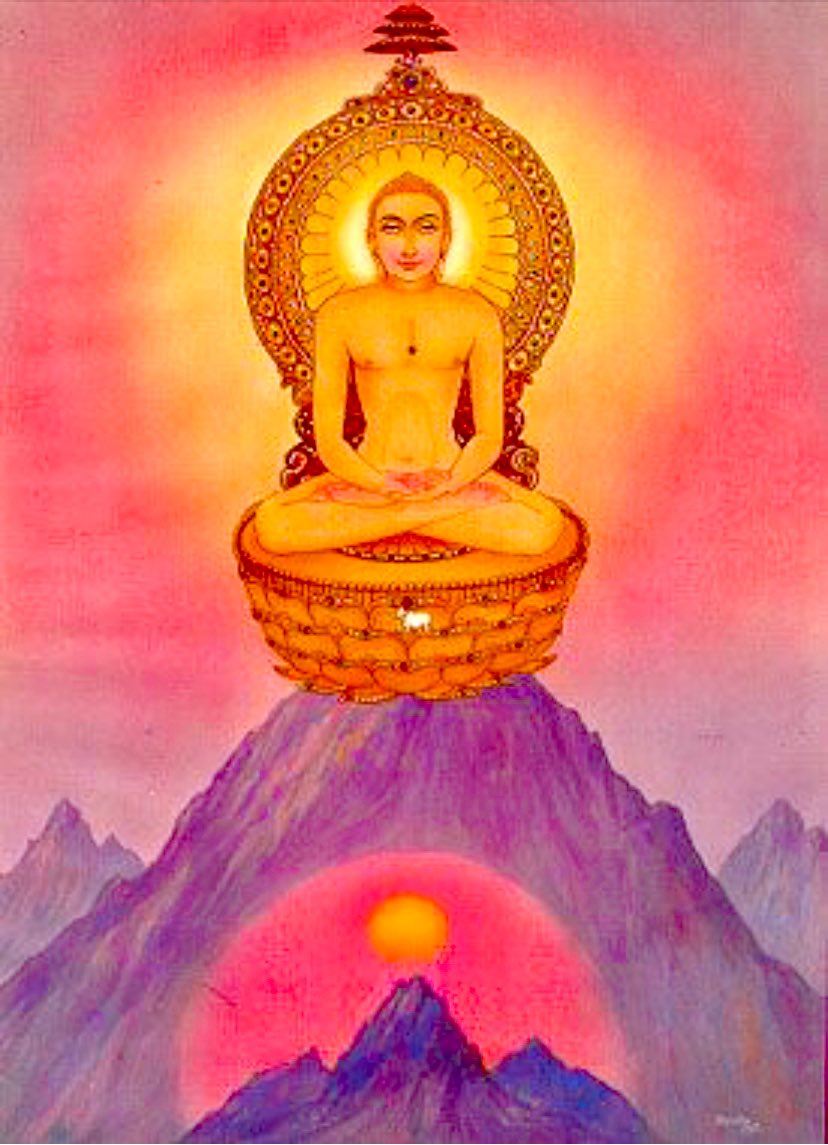In the image, a deity that exudes both Hindu and Buddhist influences is depicted seated cross-legged in a meditative pose atop a golden, intricately designed wicker throne. The deity emanates a radiant, glowing presence with a spherical halo featuring numerous ridges and concentric circles surrounding their head, symbolizing enlightenment or divine energy. A conical tree extends upward from the halo, enhancing the ethereal aura of the figure. 

The figure itself is golden-yellow and sits upon a throne that appears to float over a mountainous backdrop distinguished by deep purple hues. The primary mountain is the tallest and central, with two smaller purple mountains in the background and another smaller one in the foreground. In the middle of the deity's chest is a prominent black dot, adding a mysterious focal point.

An additional visual detail includes dual images or emblems of the sun. One right beneath the main peak, where a smaller, darker version of the deity is illustrated, replaced by a sun at the mountain's base. Below the main mountain, a glowing red orb encloses a smaller yellow sphere, intensifying the scene’s mystical atmosphere and reiterating the theme of illumination and divinity.